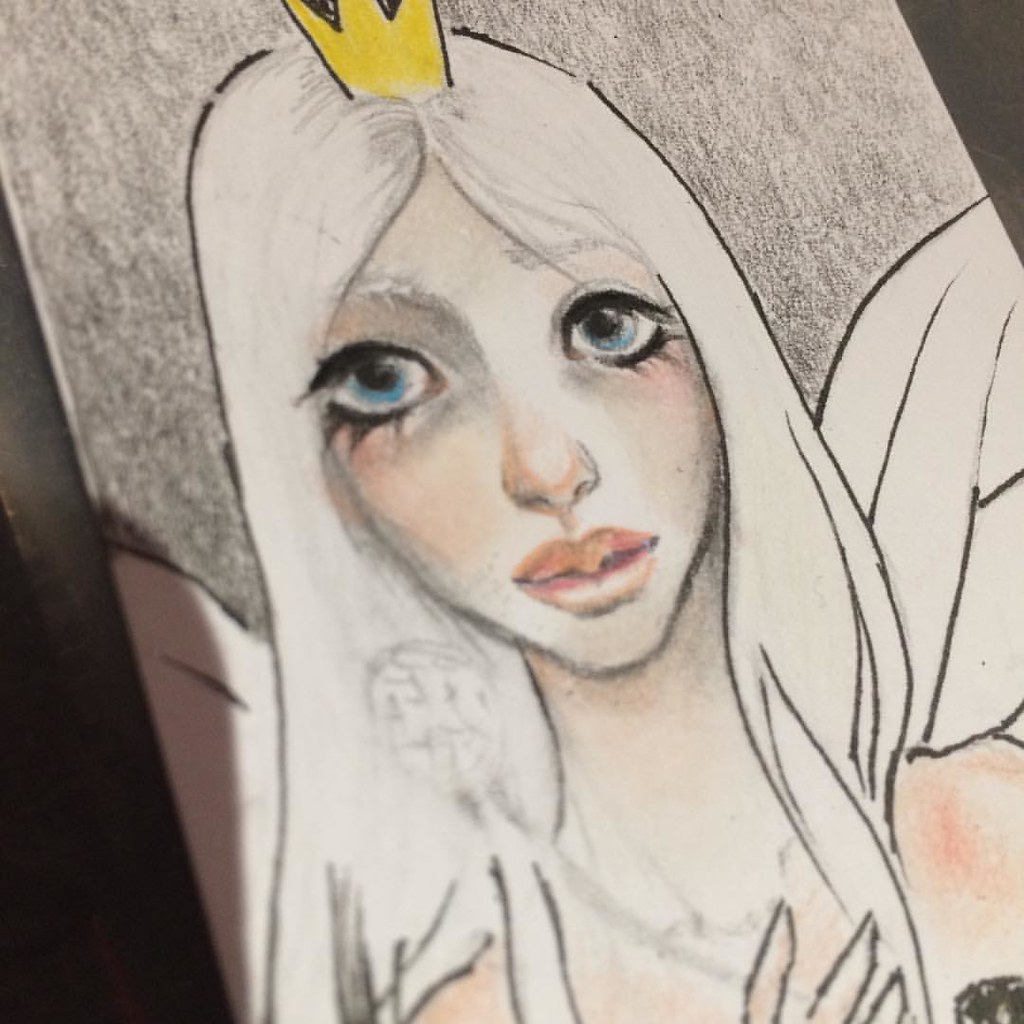In this photograph, we observe a closeup shot of a detailed artwork, potentially a drawing executed with colored pencils or pastels rather than paint. The image is taken from an intriguing angle, presenting a partial view of the piece. Dominating the composition is a female figure with strikingly large blue eyes and prominent pink lips. She is depicted with long hair and wings, both of which remain uncolored, suggesting either an unfinished aspect of the artwork or an intentional choice to keep them white. The background contrasts vividly with the figure, filled in with a charcoal-like gray hue. Notably, the female subject wears a small, gold crown atop her head. The artwork lacks any accompanying text, allowing the visual elements to convey the entirety of its narrative.